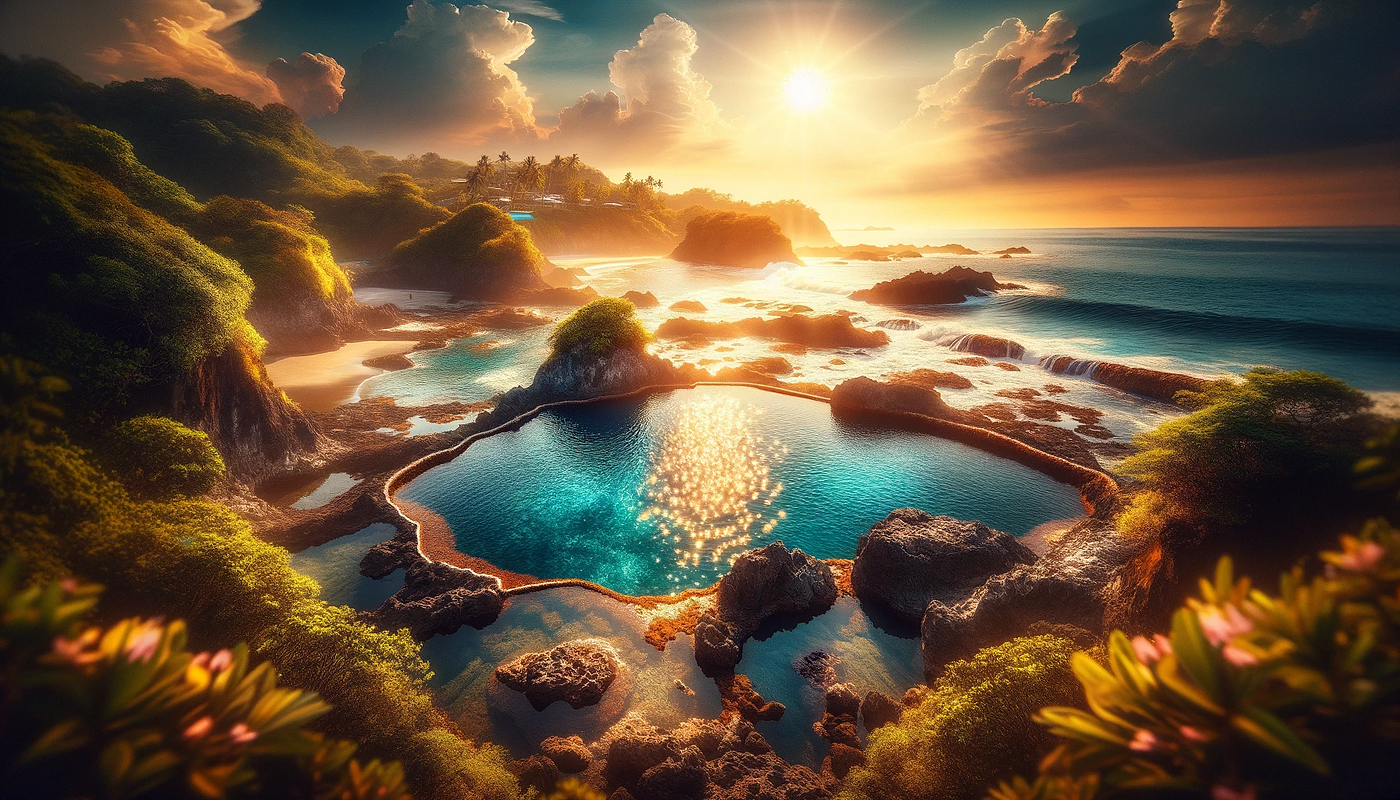This digital painting depicts a stunning futuristic outdoor scene at sunrise, characterized by a bright sun centered in the sky, casting its radiant rays upward and downward through a canvas of puffy white and golden clouds. The foreground showcases a serene pool of deep blue water, reflecting both the sky and the sun's light, surrounded by a rocky shore adorned with lush green moss and clusters of pink flowers with green leaves. To the left, green mountains and hills cascade down towards the landscape, while the right side features undulating hills and stones. In the background, imposing mountains, filled with dense greenery, shrubs, and trees, add depth to the scene. The distant horizon where the ocean meets the sky completes this idyllic and expansive setting, where rocks and greenery frame the edges, and the ocean’s waves gently lap at the shore. The entire composition exudes a harmonious blend of natural beauty and tranquility, enhanced by the vivid details and vibrant colors that illustrate the interplay between sunlight, water, and lush vegetation.